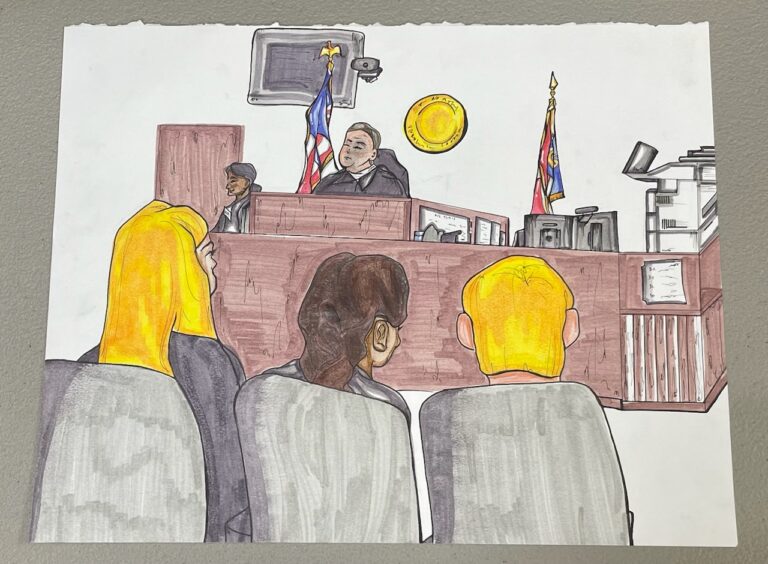The image is a photograph of a detailed courtroom painting rendered on white paper placed on a gray surface. Central to the painting, a judge is seated at a high, brown wooden desk, distinguishable by his traditional black robe. Behind the judge, a golden circular object hangs prominently on the wall. Flanking the judge are two flags: the American flag with its distinctive blue field and red and white stripes on the left, and what is likely a state flag on the right.

Adjacent to the judge on his left is a woman, contributing to the sense of judicial proceedings. In front of the judge, three individuals are seated. Notably, the person on the right and the one on the far left have golden-colored heads, while the individual in the middle has a brown-colored head. These figures, seated on chairs with green backs, appear intently focused on the judge, almost mesmerized by the proceedings. The overall scene is framed against a white backdrop, emphasizing the somber and authoritative atmosphere of the courtroom setting.